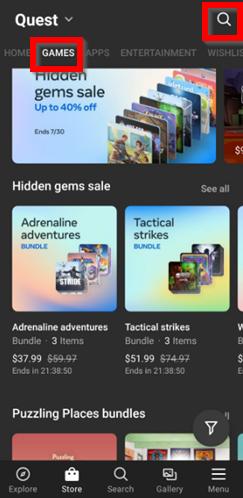In the image, the Quest website is prominently displayed. The header features the word "QUEST" in bold white letters against a black background, with the text outlined in blue. The word "games" is highlighted within a red box, drawing attention to the gaming content. Adjacent to it, a search icon is similarly outlined in a red box.

The main section showcases the "Hidden Gems Sale," with a prominent label indicating discounts of up to 40% valid until July 30. A variety of game cover images are neatly arranged, giving a preview of the collection. Below this, the text "Hidden Gems Sale See All" invites users to explore the full range of discounted games.

Among the featured bundles, "Adrenaline Adventures" is advertised, detailing that the bundle includes three items, now priced at $37.99, down from the original $59.97. A countdown timer shows the sale ending in 21 hours, 38 minutes, and 50 seconds. Similarly, "Tactical Strikes" includes three items at a discounted price of $51.99 from $74.97, with the same time remaining for the sale.

Further down, the "Puzzling Places" bundle offers even more options for users. The footer of the website provides navigation options including "Explore," "Store," "Search," "Gallery," and a "Menu" button, allowing users to easily access different sections of the site.